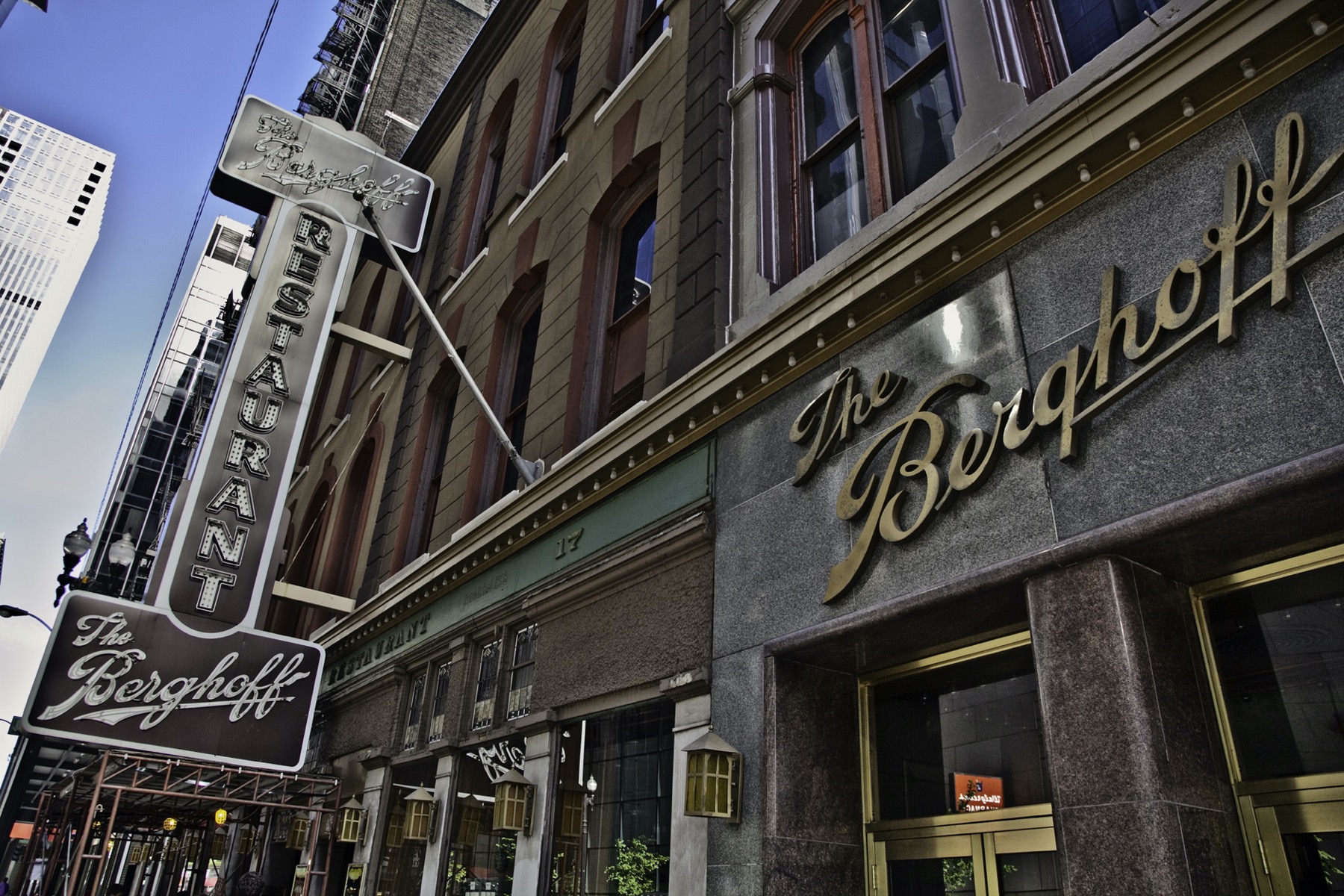In the vibrant downtown area, amid the daylight and clear blue sky, stands an impressive photograph showcasing various storefronts set against towering residential buildings. Dominating the foreground from the pedestrian perspective on the sidewalk is a large, brown multi-story building with expansive windows. Notable on the ground level is the eye-catching storefront of "The Berqhoff," a renowned establishment whose name is elegantly displayed on a large sign. This sign, accented in an aged metal that once gleamed golden, hangs above the entrance flanked by two large glass doors with gold-colored frames, set into a facade of sleek, dark black marble tiles. Adjacent to this, another broad black signboard prominently reads "Restaurant The Berqhoff." Although the golden hues show signs of rust and wear, the grandeur of the sign remains. In the background, newer, soaring white skyscrapers further amplify the dynamic juxtaposition of the old and the new. The composition, enhanced by the bright sunny day, beautifully captures the historic charm and urban vibrancy of this bustling downtown street.